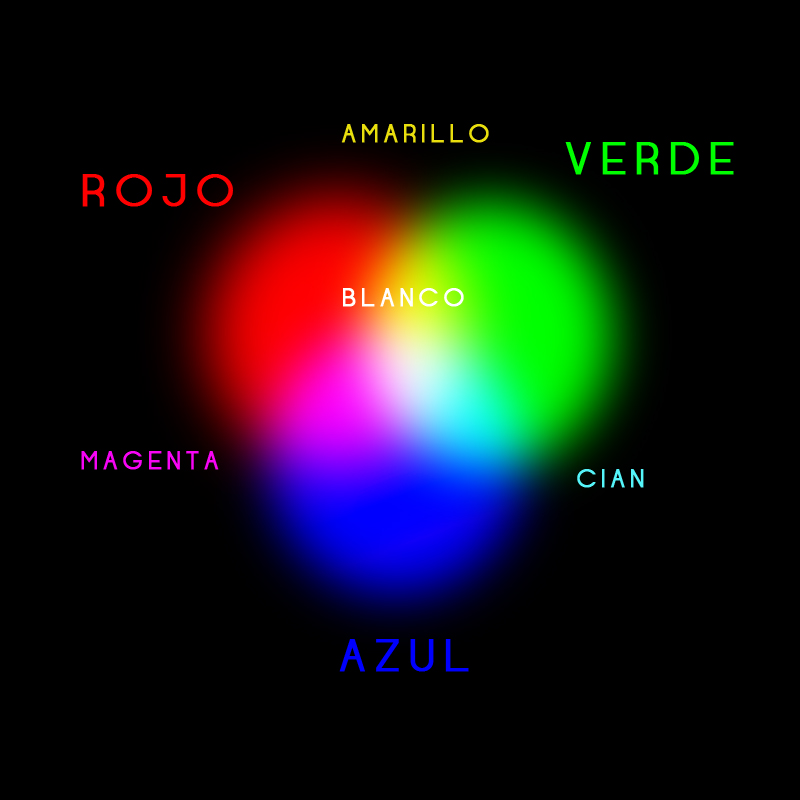This is a computer-generated image of a color chart with a black background. At the center, there are three intersecting circles of different colors: a red circle on the left labeled "Rojo," a green circle on the right labeled "Verde," and a blue circle at the bottom labeled "Azul." Where the circles intersect, they create additional colors: yellow labeled "Amarillo" above the intersection of the red and green circles, light blue labeled "Cyan" next to the intersection of the green and blue circles, and purple labeled "Magenta" next to the intersection of the red and blue circles. In the central intersection of all three circles, it says "Blanco" in white, representing white. The words in Spanish are color-coded to match the respective colors they describe.